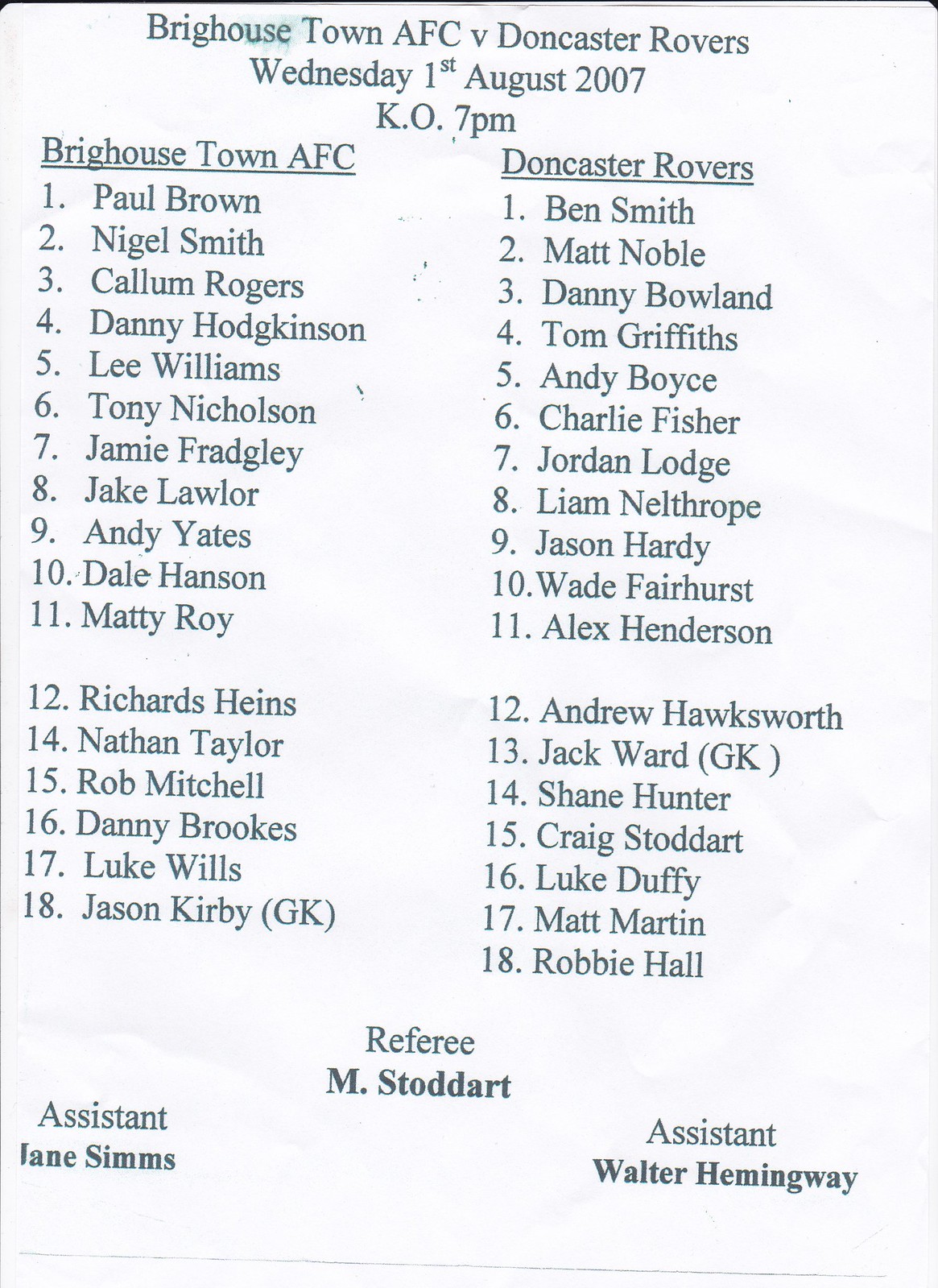This vertical rectangular image resembles a page from a soccer match program with a light blue background and black text. At the top, the heading reads, "Brighouse Town AFC versus Doncaster Rovers, Wednesday, 1st August, 2007, KO 7 PM." Below this, the page is divided into two columns. The left column is labeled "Brighouse Town AFC" and lists 11 player names, followed by a space and names for players numbered 12 through 18. The right column is labeled "Doncaster Rovers," also listing 11 player names, followed by a space and names for players numbered 12 through 18. At the bottom of the page, the referee is listed as M. Stoddard. On the bottom left side, the assistant referee is named Lane Sams, and on the bottom right side, the assistant is Walter Hemingway.